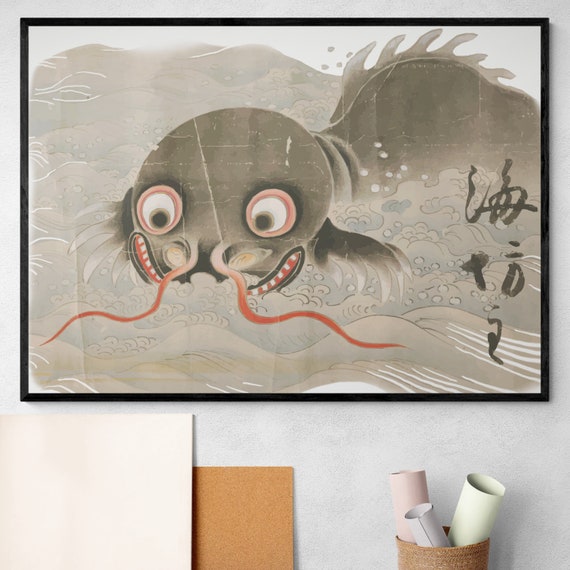The artwork features an exquisitely detailed Japanese pen and ink, possibly watercolor, drawing that appears to be quite traditional and potentially from the 1800s or earlier. Framed in a thin black frame, the piece showcases a playful yet ancient-looking sea monster with large eyes and red tendrils sprouting from its face. The creature, predominantly in shades of gray and red, emerges amid crashing waves, its toothy smile lending the overall scene a whimsical yet enigmatic feel.

Accompanying the image, Japanese or Chinese characters, likely the artist's signature, embellish the right side of the piece, adding an authentic touch to the traditional aesthetic. Below the frame, a wooden bowl contains three rolled-up papers in muted shades of green, purple, and pink. Additionally, leaning against the lightly gray-colored wall under the artwork, there is a white canvas and a wooden piece, contributing to a creatively cluttered yet organized display.